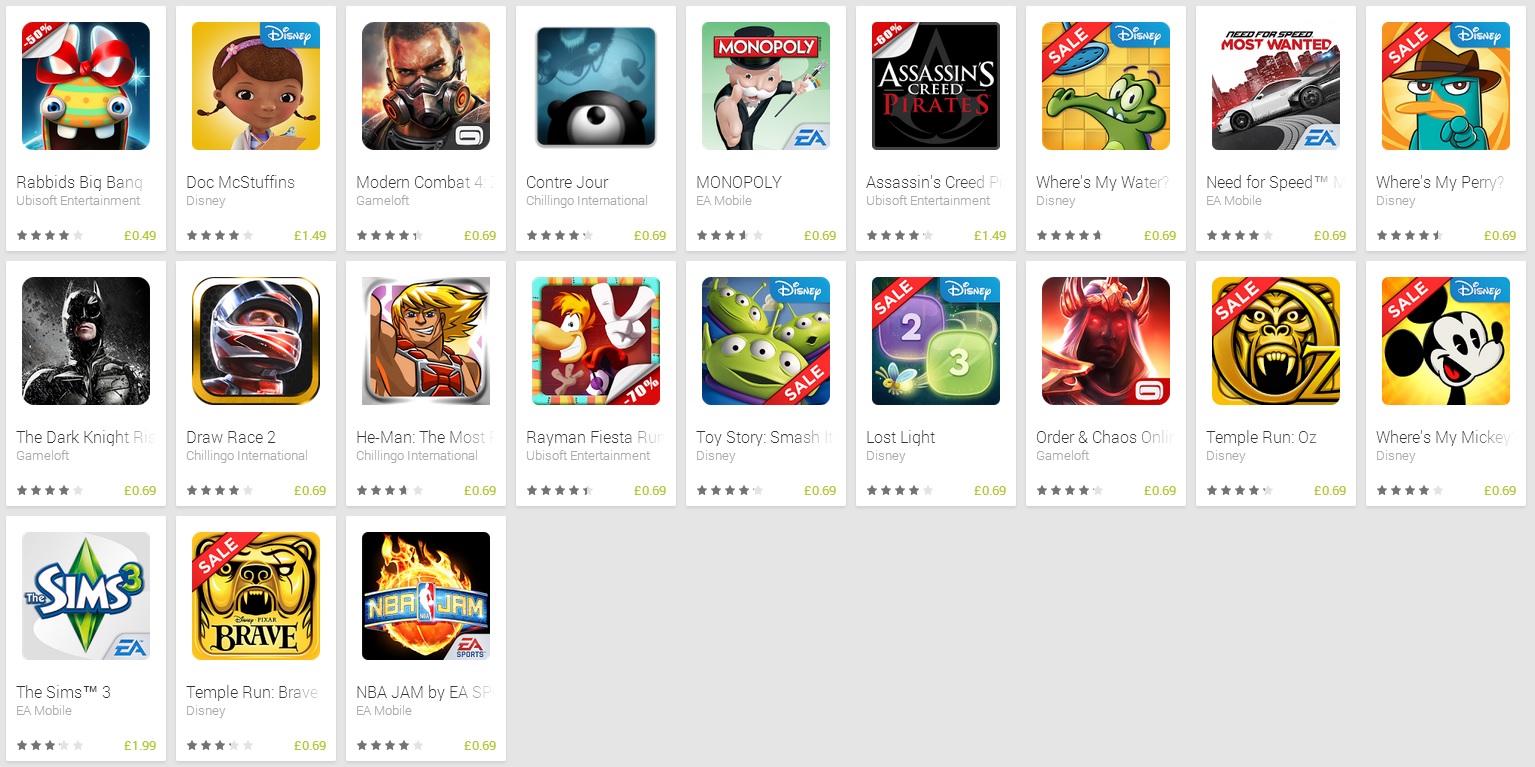The webpage features a light blue background, structured into three horizontal rows showcasing various games. Each game is encapsulated in a small white square that highlights the game’s cover image along with its star rating and price. The cover images predominantly display vibrant cartoon artwork.

- **Rabbids Big Bang:** Featuring a frenzied rabbit cartoon face, this game stands out with its distinct crazed expression.
- **Doc McStuffins from Disney:** Illustrates a joyful black female doctor. She is depicted wearing a lab coat and holding a clipboard with a radiant smile.
- **Modern Combat 4:** As part of the lineup, this game features intense action themes, though specific imagery is not detailed.
- **Contre Jour by Chillingo International:** This game’s cover art is more abstract, focusing on unique, shadowy figures.
- **Monopoly:** Highlights the classic board game, likely with familiar elements like Rich Uncle Pennybags.
- **Assassin's Creed Pirates:** Showcases swashbuckling pirate adventure themes tied to the famous franchise.
- **Disney's Where's My Water:** Features a cheerful cartoon alligator, central to the game’s water puzzle mechanics.
- **Need for Speed:** Focused on high-speed racing, though the cover specifics are unspecified.
- **Where's My Perry?:** Depicts an angry cartoon bird wearing a detective hat, known for its engaging puzzle gameplay.
- **The Dark Knight:** Likely features Batman themes, inferred from the name, though not explicitly described.
- **Draw Race 2:** This title suggests racing mechanics but lacks specific visual context.

The description highlights a wide array of games within the layout, each presented with appealing and colorful visuals designed to capture the viewer’s interest.